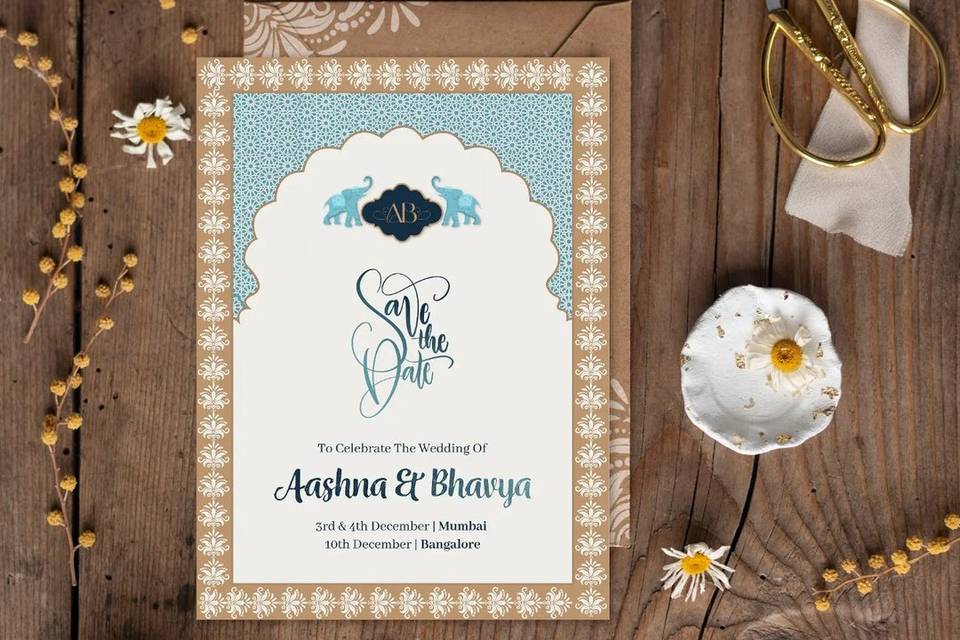This image is a detailed top-down photograph of a wedding invitation laid flat on a wooden tabletop. The background showcases various decorative elements, including scattered flower heads, branches, and the golden handles of a pair of scissors partially visible at the top right corner. 

The invitation itself features a mauve border adorned with an intricate white floral design. At the top of the invitation, two light blue elephants with their trunks raised frame a golden monogram displaying the initials "AB." Centrally, the phrase "Save the Date" is elegantly scripted in ornate cursive lettering. Beneath this, in clear but smaller letters, it reads, "to celebrate the wedding of Ashna and Bhavya," with their names prominently highlighted in larger text.

At the bottom of the invitation, the dates and locations for the wedding festivities are listed: "3rd and 4th December, Mumbai, 10th December, Bangalore," indicating multiple celebratory events likely spanning a weekend and a subsequent date. The overall design and color scheme, including the tan-colored paper with contrasting dark and light blue lettering, suggest a sophisticated and cultural aesthetic, hinting at a traditional Indian wedding.